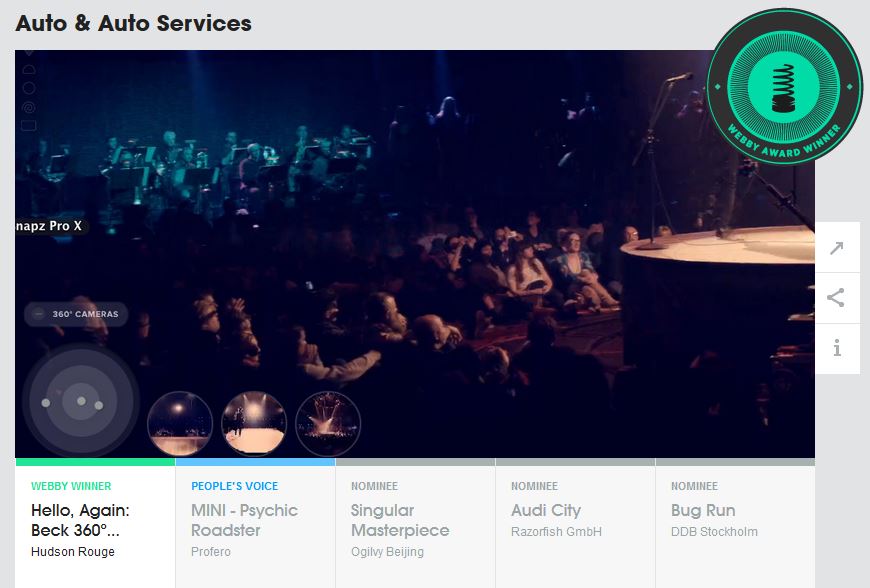Screenshot Description:

The screenshot appears to be from a webpage related to automobile services, as indicated by the title "Auto and Auto Services" located at the top-left corner. The main feature of the screen is a large photo that occupies about two-thirds of the space. This photo displays a crowd of people seated and watching a concert; however, the performer on stage is not visible.

Below the photo, there are several buttons that seemingly allow users to navigate to different sections or items. From left to right, the buttons display the following labels: "Webby Winner," "Hello Again Beck 360," "Hudson Rouge," "People's Voice," "Mini Psychic Roadster," "Nominee Singular Masterpiece," "Nominee Oddy City," and "Nominee Bug Run." These buttons span the width beneath the large central photo.

The overall design includes a few additional navigational elements, with a navigation bar on the right side. The top of the page has a light gray header, and both the sides and bottom of the page feature a gray border, with the bottom being a lighter shade.

In summary, the webpage layout includes a prominent photograph of a concert audience, navigation buttons for various sections or awards, and thematic borders, all under the main heading "Auto and Auto Services."